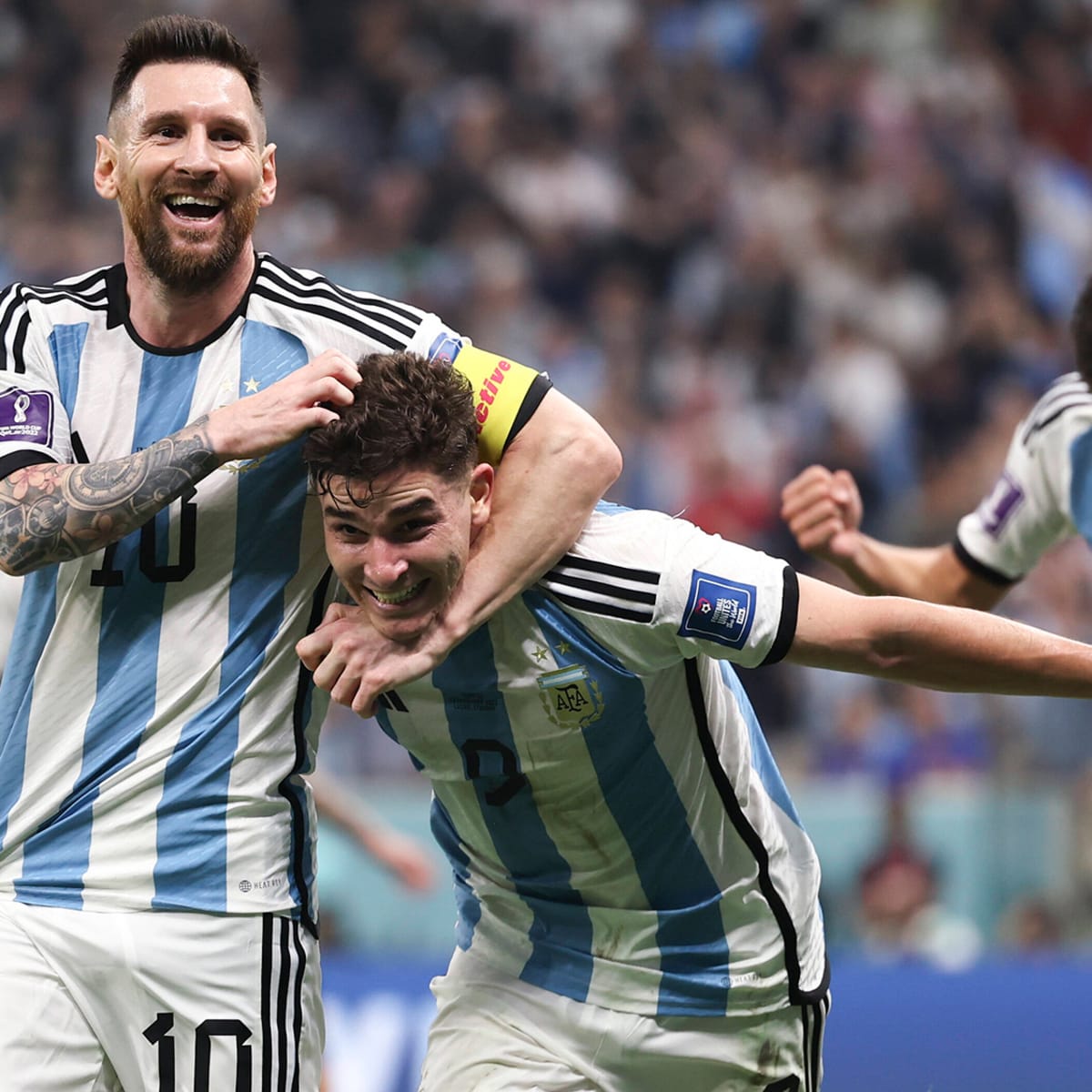This image captures a close-up of two jubilant soccer players mid-celebration on the field, possibly after scoring a goal. Both athletes are dressed in light blue and white striped jerseys and white shorts. The player on the left, who closely resembles the famous Messi and wears the number 10 jersey, has a short beard and spiky hair. He is playfully holding his teammate, whose jersey number is obscured, in a lighthearted headlock, ruffling his hair with a playful gesture. The second player, with short wavy hair and no beard, grins broadly. Their joy is unmistakable, mirrored by the blurred but densely packed stadium filled with cheering fans. Another player's fist, likely from the same team, is visible on the edge of the frame, adding to the moment's excitement. The scene is vibrant, full of energy, and captures the camaraderie and elation experienced in the heat of the game.